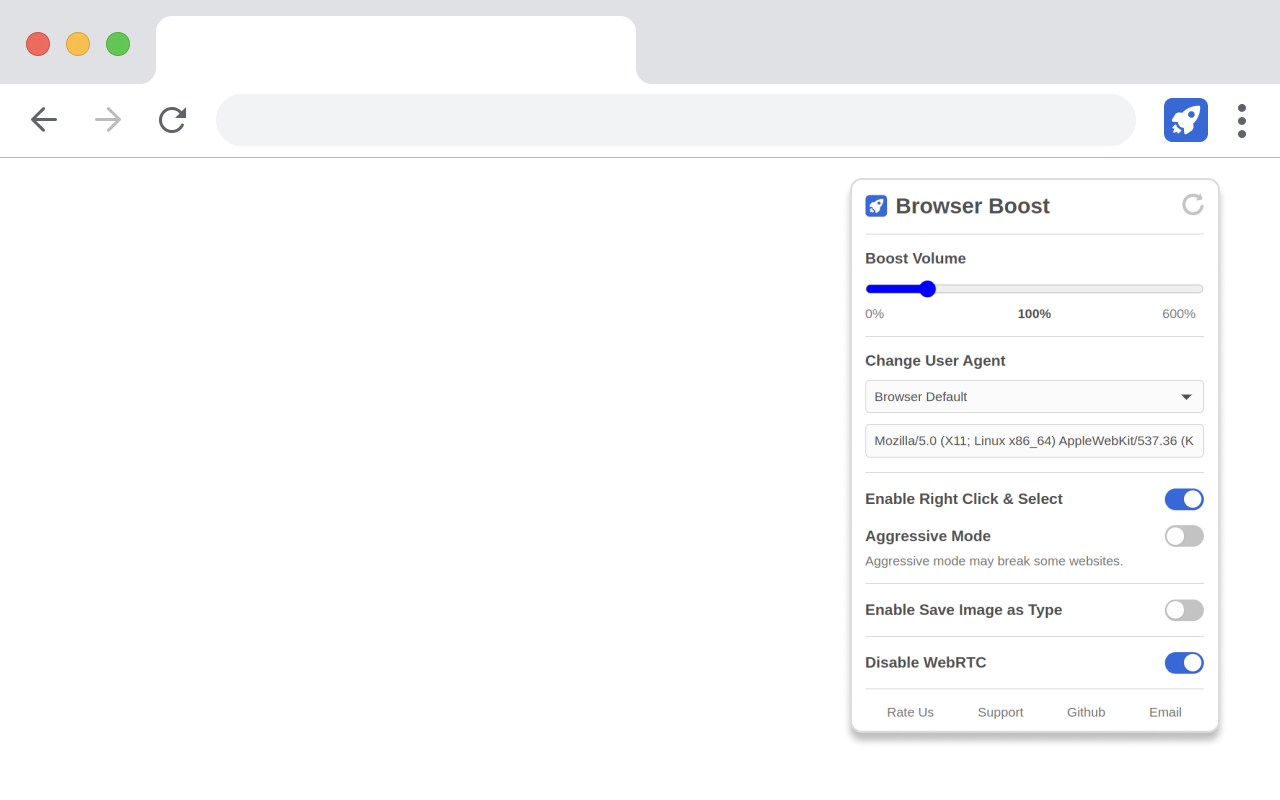This image depicts an internet browser window, specifically Google Chrome, as indicated by the presence of the distinctive red, yellow, and green dots in the upper left-hand corner. The address bar and search bar are both empty, signaling that no specific URL or search query is currently active. Spanning across the screen is a submenu titled "Browser Boost." This submenu provides several adjustable features: a boost volume control, an option to change the user agent, and four toggle switches. The toggle switches offer the following functionalities: "Aggressive Mode," "Enable Right-Click and Select," "Enable Save Image As Type," and "Disable WebRTC." Each of these toggles allows the user to customize their browsing experience by enhancing control, accessibility, and security.